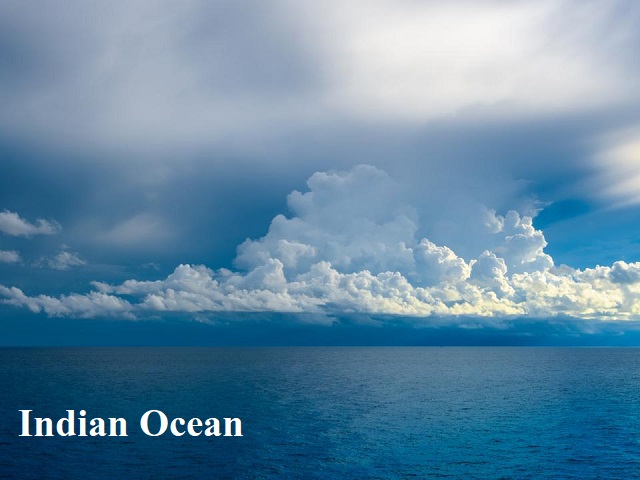This photograph captures the expansive and serene beauty of the Indian Ocean as indicated by the text in white letters in the lower left-hand corner. The lower quarter of the image features a vast, calm ocean with a smooth surface, extending to the horizon where it meets a clear blue sky. The sky dominates the upper three-quarters of the photo, showcasing a diverse array of cloud formations. Just above the ocean, the sky is a deep blue, transitioning into a band of thick, fluffy white clouds. Higher up, the clouds become more diffuse and fog-like, almost resembling the plume of a volcanic eruption, with soft sunlight attempting to break through, casting subtle shadows on the water below. The overall palette of the image is a soothing mix of blues and whites, creating a tranquil and evocative scene.